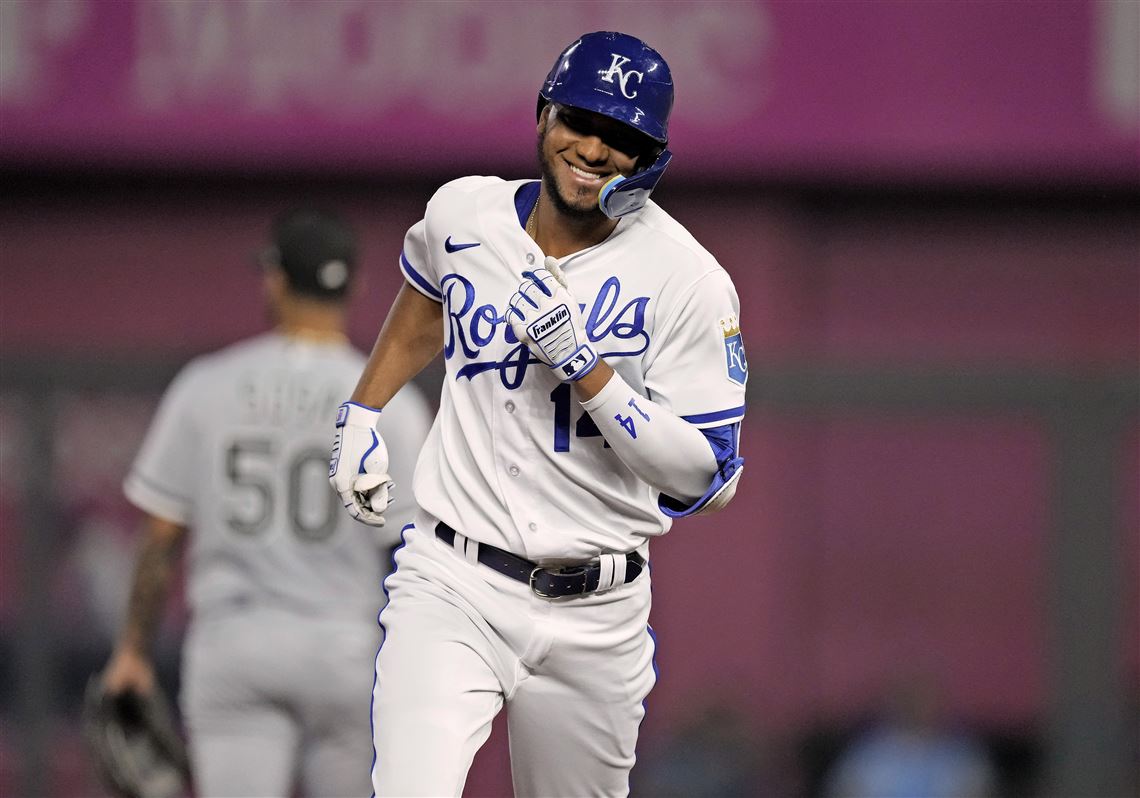The photograph captures an African American male athlete, likely a Major League Baseball player, in the middle of running the bases. He is adorned in a Kansas City Royals uniform that consists of a white short-sleeved jersey with the word "Royals" elegantly scripted in blue on the front, adorned with a blue Nike swoosh on the right shoulder. The player’s ensemble includes white pants accented with blue pinstripes on the sides, secured by a black belt, and he wears matching white and blue gloves. His blue batting helmet prominently features the white letters "KC" at the front. The athlete is joyfully smiling with his mouth open, adding a sense of exuberance and energy to the image.

In the background, another player in a gray uniform with the number 50 is partially visible but out of focus, likely indicating motion or depth of field. This player is equipped with a black glove and a cap, contributing to the action-packed ambiance. Additionally, the largely blurred backdrop reveals a pinkish or purplish wall, the details of which remain indistinct, offering a contrasting background hue to the vivid scene.